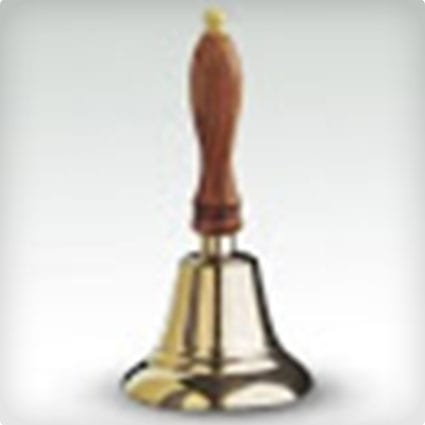This image is a grainy and slightly blurry color photograph featuring a single object: a hand bell. The background varies in descriptions but leans towards a solid, white or light gray/tan color. The bell itself is prominently gold with a shiny surface that reflects some black shadows, suggesting a glossy texture despite the image's low quality. The bell is approximately an inch and a half to two inches in length and width. The handle is wooden, relatively small, measuring about a half-inch in diameter and roughly two inches long. At the top end of the handle, there is a noticeable yellow tip, which could be plastic or wood. The bell is positioned in the center of the image, standing upright with the handle facing upwards. There are no other objects or text in the picture, and the bell appears to be in good condition despite the poor image quality, which hints at an indoor setting where such a bell might typically be used.